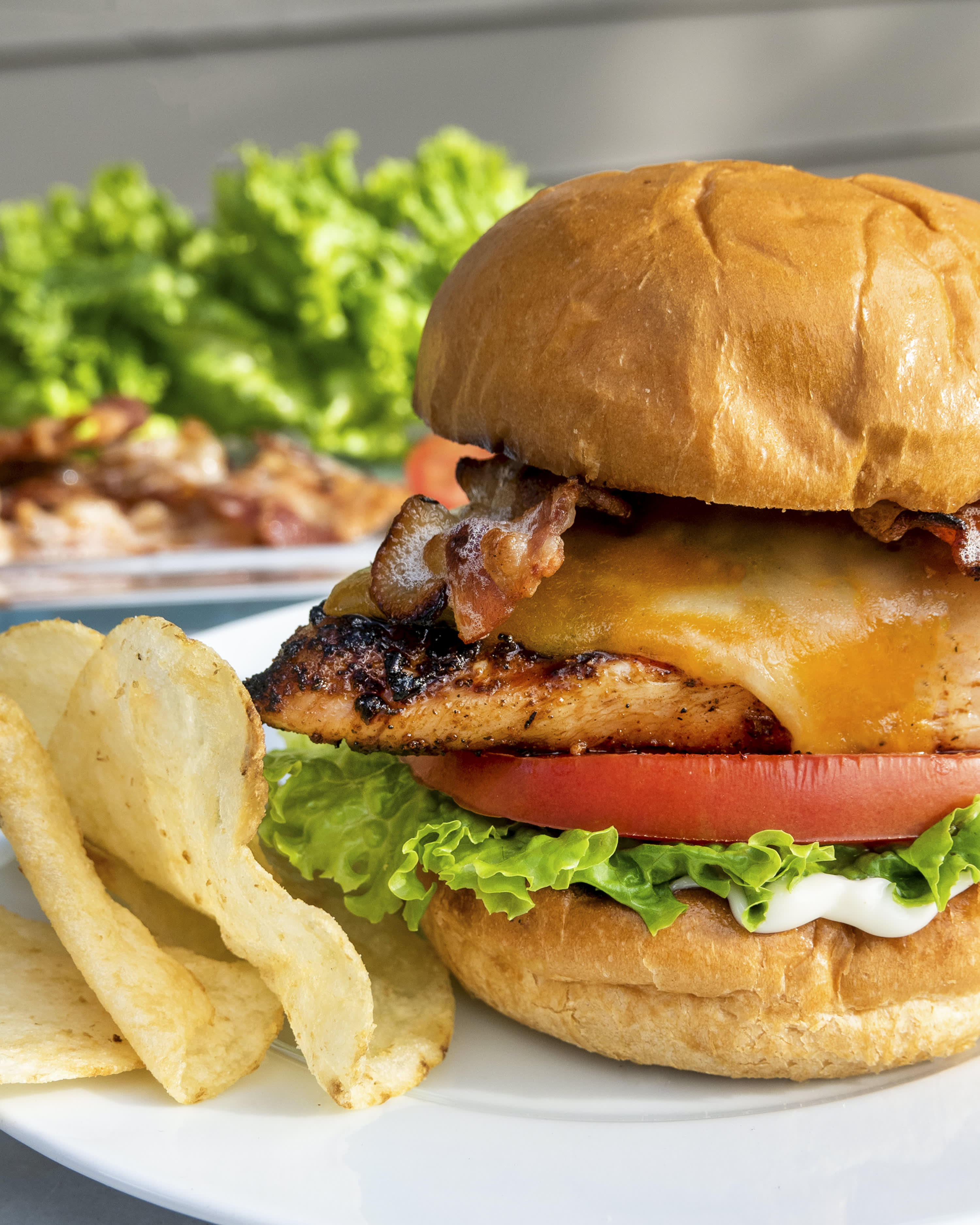This close-up shot features a mouthwatering chicken sandwich on a white plate, accompanied by a side of light and crispy potato chips. The sandwich is meticulously composed: a fluffy, toasted brown bun charred at the edges; layers of crispy bacon and a slice of melted dark yellow cheddar cheese draped over a char-grilled chicken breast; all resting atop a vibrant red tomato and a bed of fresh green lettuce. A tantalizing dollop of mayonnaise spills over the edge of the bottom bun. To the left of the sandwich, three delectable light yellow potato crisps lie invitingly. The background, artfully out of focus, reveals a glass plate laden with more crispy bacon and another scattered plate of lettuce, adding depth to this appetizing scene. The overall presentation could easily grace a culinary advertisement.